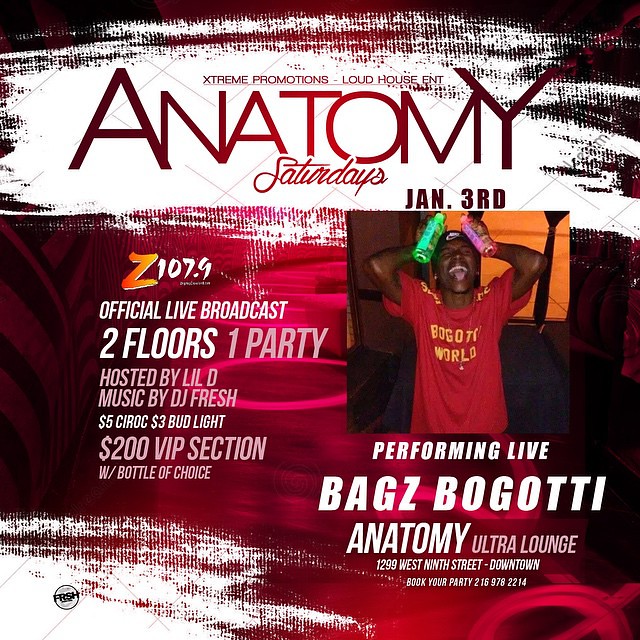The promotional poster, predominantly showcasing a dark red and black theme interspersed with a splash of white paintbrush-like designs, advertises an upcoming musical performance event. At the top, against a white background, it reads in small letters: "Extreme Promotions, Loud House ENT." Below it, "Anatomy" is boldly highlighted, followed by "Saturdays" and "January 3rd" in a similar prominent font. Adjacent to the text is an image of a man in a red t-shirt, eyes closed and mouth open, holding two bottles up by his head. This image is brightly illuminated, forming the focal point of the poster. 

Underneath the image, it states in large white letters, "Performing Live: Bogoty," alongside details of the venue: "Anatomy Ultra Lounge, 1299 West 9th Street Downtown. Book Your Party: 216-978-2214." 

On the left side, further details highlight a "Z107.9 Official Live Broadcast. Two Floors, One Party. Hosted by Lil D. Music by DJ Fresh," including drink specials: "$5 Ciroc, $3 Bud Light" and a "$200 VIP Section with Bottle of Choice." The entire poster is bathed in bright, shiny colors, contrasting against a dark red and pinkish backdrop, giving it a vibrant, lively appearance.